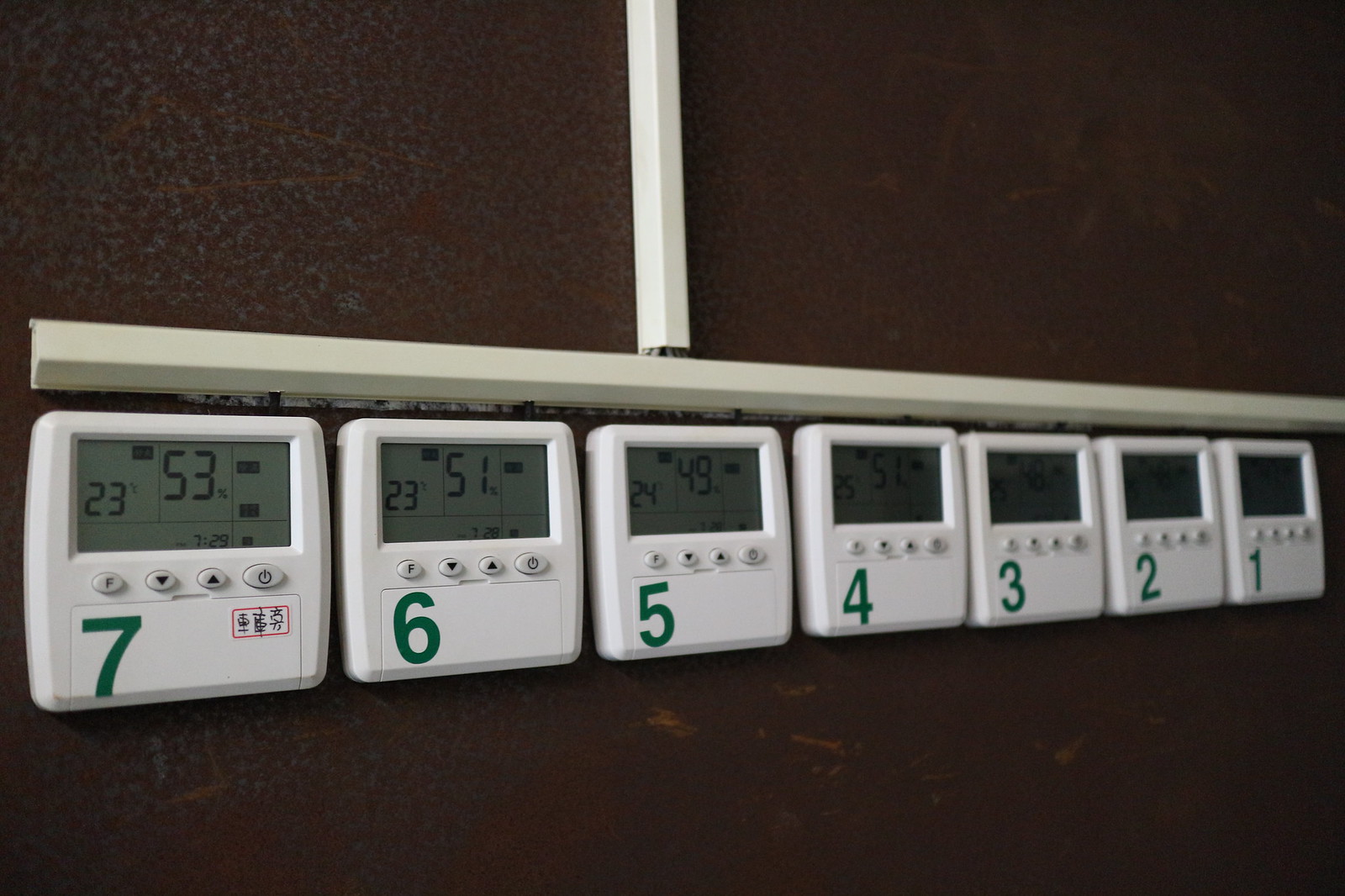In the photo, the background features a burgundy hue interspersed with patches of gray. The focus is on a grid-like structure, which seems to be either a window or a wall, divided by vertical and horizontal lines. Beneath the horizontal line, there are seven small white square boxes arranged in a row. Each box is numbered sequentially in green, starting from the left with 7, followed by 6, 5, 4, 3, 2, and ending with 1 on the right.

Above the numbers on each box, there are four small buttons. The buttons include a power button, an up button, a down button, and a button marked with a black "F". Within each box, the display shows various numbers: 

- Box 7 displays "2353".
- Box 6 displays "2351".
- Box 5 displays "2449".
- Box 4 displays "2551".
- Box 3 partially displays numbers, showing "46" and "25".
- The numbers on boxes 2 and 1 are not visible.

These boxes resemble thermostats, and they are evidently the central focus of the image.